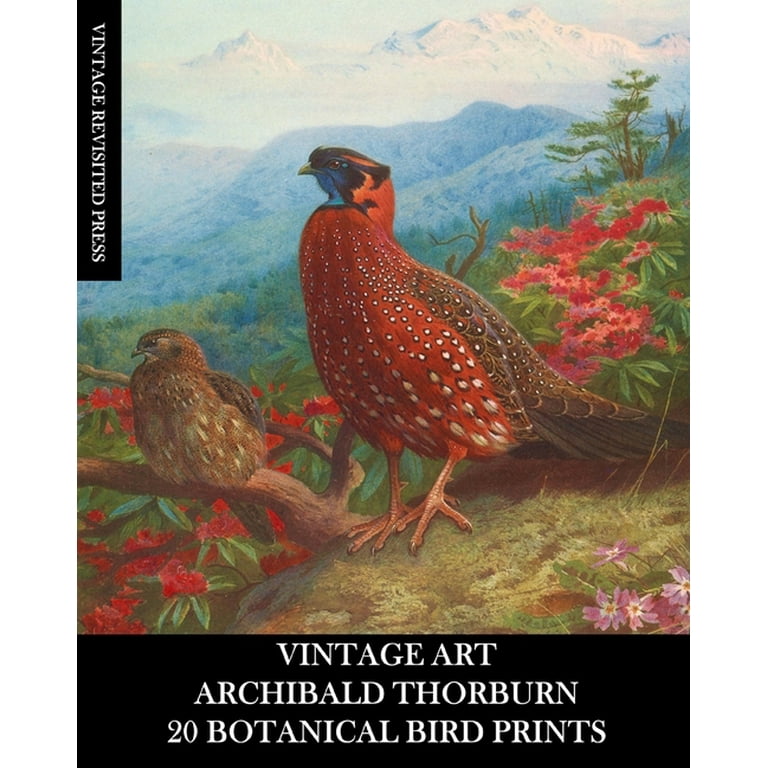This vibrant advertisement for "Vintage Art" by Archibald Thorburn showcases a lushly detailed illustration of two birds amidst a richly layered natural backdrop. In the upper left, rotated 90 degrees clockwise, is a black rectangle with white text that reads "Vintage Revisited Press." Along the bottom, another black rectangle displays in white text, "Vintage Art, Archibald Thorburn, 20 Botanical Bird Prints." At the center of the image, two birds are prominently featured: the larger bird, perched on a grassy mound, has striking red feathers adorned with white spots, a blue face with a distinct black outline, and brown feathers on its back and tail. Its large orange feet are firmly planted in the grass below. The smaller bird, seated on a branch to the left, is more modestly colored with brown feathers and white speckles. The scene is further enlivened with bright red and pink flowers, green vegetation, and a dramatic background featuring lush green hills, dense woods, and snow-capped mountains against a blue sky. This vividly detailed print captures the essence of Thorburn's exquisite botanical bird artistry.